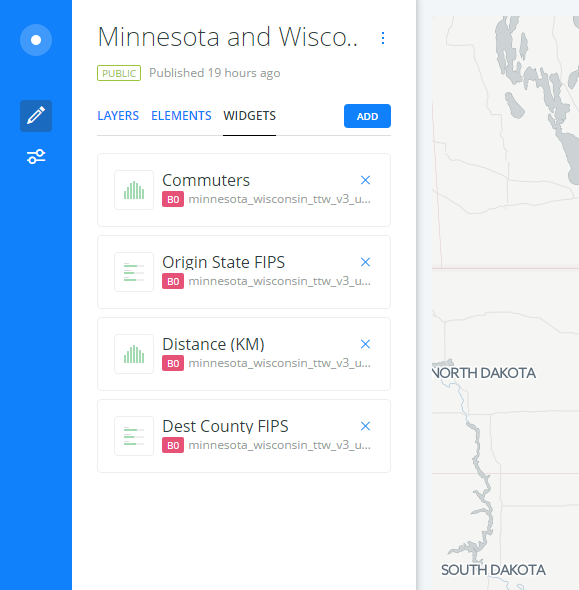The image is a screenshot featuring a detailed interface. On the left side of the screenshot, there is a vertical blue bar. At the top of this bar, there is a white circle with a lighter white or light blue outline. Beneath this circle, there are two icons: a pencil icon and an icon that resembles a line with circles on each end. Below these icons, text that partially reads "Minnesota and Wisco..." is visible, suggesting it is cut off.

On the right side of the screenshot, there is a gray-colored map displaying various geographical features, including rivers and borders. The map is partially obscured at the top, but the bottom section clearly shows the labels "North Dakota" and "South Dakota," providing orientation.

In the central section of the screenshot, there is a header with three tabs labeled "Layers," "Elements," and "Widgets." The "Widgets" tab is currently selected, indicated by a black underline, while the other two tabs are in blue. To the right of the tabs, there is a blue "Add" button.

Below the header, there are four distinct rectangles, each containing different data fields: "Commuters Origin," "State Fits," "Distance (in kilometers)," and "Destination or Dust County Fits." Each of these rectangles has a small square logo on the left side and a blue "X" button on the right side.